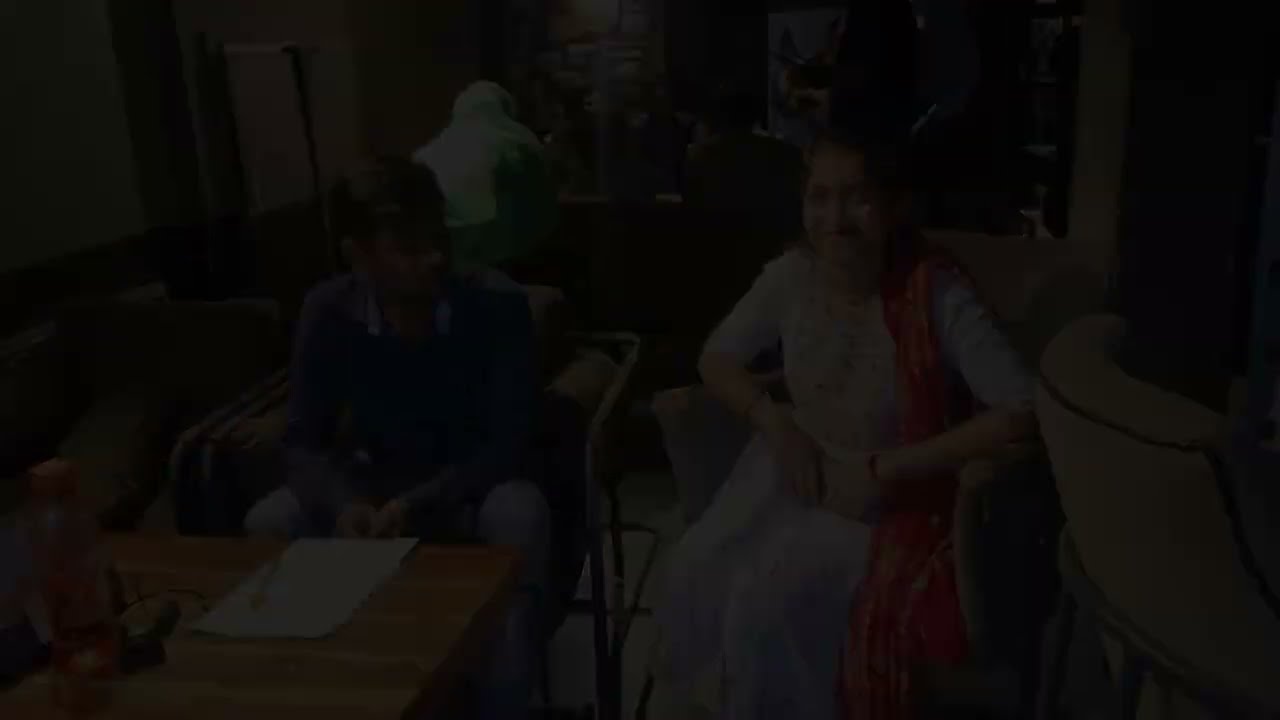This image is extremely dark, almost as if a heavy black filter has been applied, making it very difficult to discern specific details. In the foreground, there appear to be two people sitting next to each other. The person on the right is a woman, possibly South Asian, wearing a floor-length dress which might be light pink or white, accompanied by a long, red or orange scarf draped over her shoulder. She is smiling and looking directly at the viewer, her hands placed on her lap, and she seems to be wearing a bracelet on her left wrist. Next to her on the left is a man with dark hair, dressed in a long-sleeved, dark-colored, possibly blue or gray, shirt, and light-colored pants, potentially blue jeans. In front of him is a wooden desk or table with a piece of paper and a pen or pencil on it. To the far right, there is an additional, possibly empty, chair upholstered in cream-colored fabric with a black trim. The background reveals a few more figures, albeit very indistinctly, due to the dimness of the image.